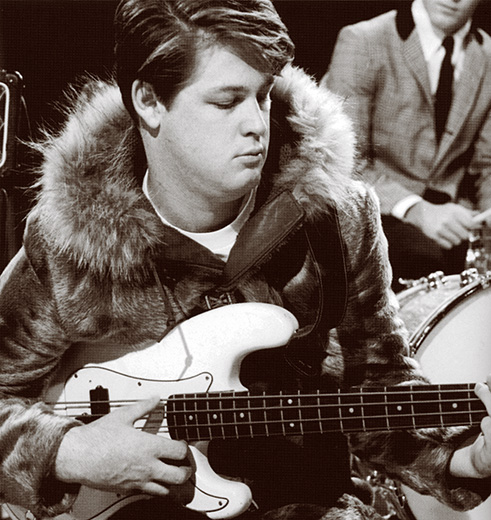This black and white photograph captures a detailed scene of a young, white male musician with dark, medium-length hair, combed over and parted on the side. He is seated and engrossed in playing a white-bodied electric bass guitar, closely examining the fretboard as he plays. The musician is adorned in a distinctive black fur coat with a hood, trimmed with fluffy, whitish fur. Positioned to the right and slightly behind the bassist is another man, likely the drummer, who is dressed formally in a white button-down collared shirt, a black tie, and a gray suit jacket with a black collar. The drummer is seen mid-action, holding drumsticks and partially obscured by a large bass drum. Both individuals are engaged in their music, contributing to what appears to be a live music event. The monochromatic composition emphasizes the texture and contrast in their attire and instruments, adding a timeless quality to the image.